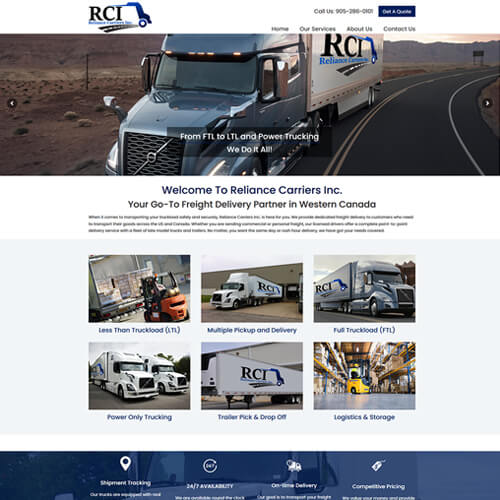The image showcases a webpage for Reliance Carriers Inc. (RCI), a freight delivery company. At the top, the page features the RCI blue logo along with a "Call Us" option beside a prominent blue button. Various navigation sections are visible, including "Our Services," "About Us," and "Contact Us."

Central to the webpage is an image of a large blue truck with the RCI logo emblazoned on the side and a white trailer. Beneath this truck, the text reads "From FTL to LTL. Power Trucking. We do it all." Additionally, a welcoming message states, "Welcome to Reliance Carriers Inc., Your go-to freight delivery partner in Western Canada."

The page is filled with illustrative images of different trucks bearing the RCI logo, highlighting the services offered: "Less Than Truck Load," "Multiple Pickup and Delivery," "Full Truck Load (FTL)," "Power Only Trucking," "Trailer Pick and Drop Off," and "Logistics and Storage."

Towards the bottom of the page, there are sections dedicated to "Shipment Tracking," "24/7 Availability," "On-Time Delivery," and "Competitive Pricing," each accompanied by relevant images, such as a white price tag for competitive pricing. The webpage is predominantly white with black text, and it includes various images of trucks, reinforcing the company's extensive service offerings.